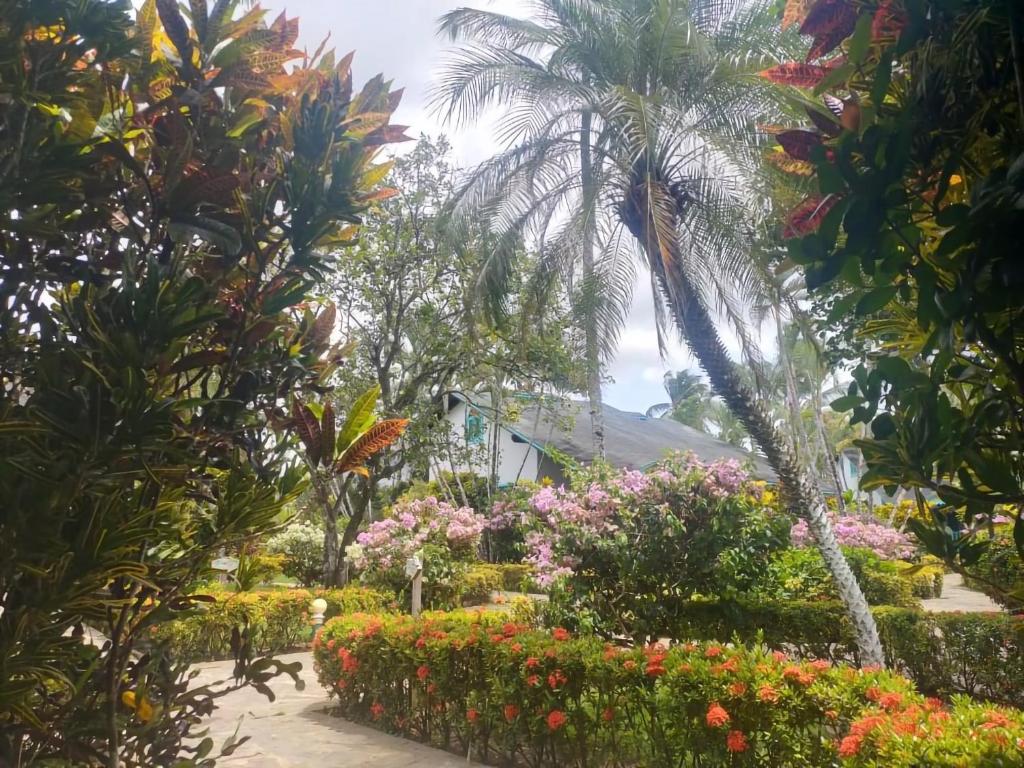A picturesque scene of a home's exterior, showcasing a charming white house adorned with a large, sloped gray roof. The setting, possibly either the front or backyard, features a gently curving paved walkway leading up to the house, surrounded by lush green bushes dotted with vibrant red flowers. To the side, a majestic palm tree stands tall, accompanied by a cluster of bushes blooming with delicate light pink flowers. The backdrop is a serene sky, painted in soft hues of light blue and scattered with a few fluffy white clouds, adding to the tranquil ambiance of the yard.